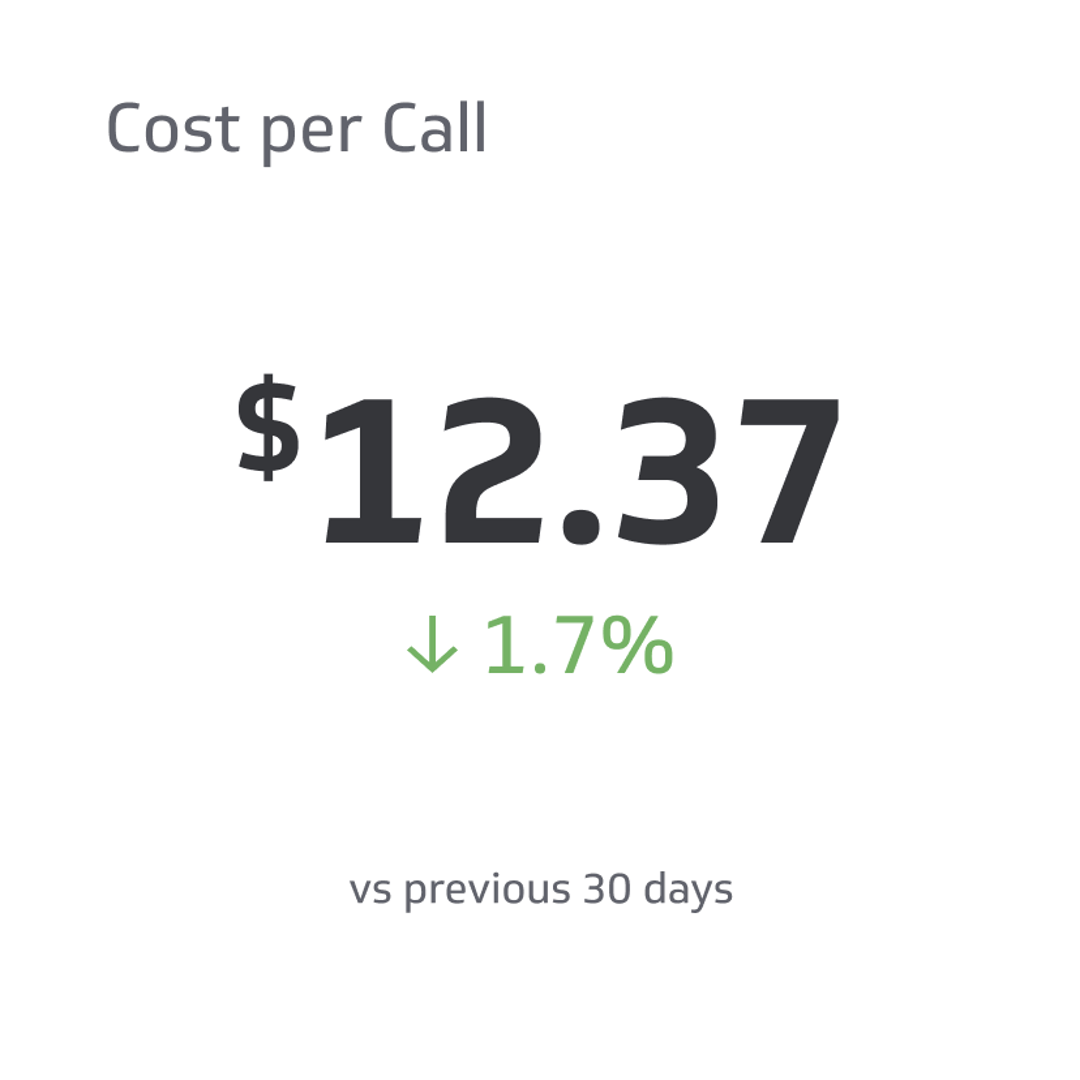A detailed screenshot capturing a performance metric: the upper left corner prominently features the label "Cost per Call." Dominating the center of the screen, in bold black numbers, the current cost per call is displayed as $12.37. Directly beneath this, a green arrow pointing downward signifies a positive trend, accompanied by a green "1.7%" indicating a 1.7% decrease. Further below, in smaller black letters, the text "versus previous 30 days" provides context, comparing the current figure to the past month. This is all presented against a clean and minimalistic background, emphasizing the key data points.